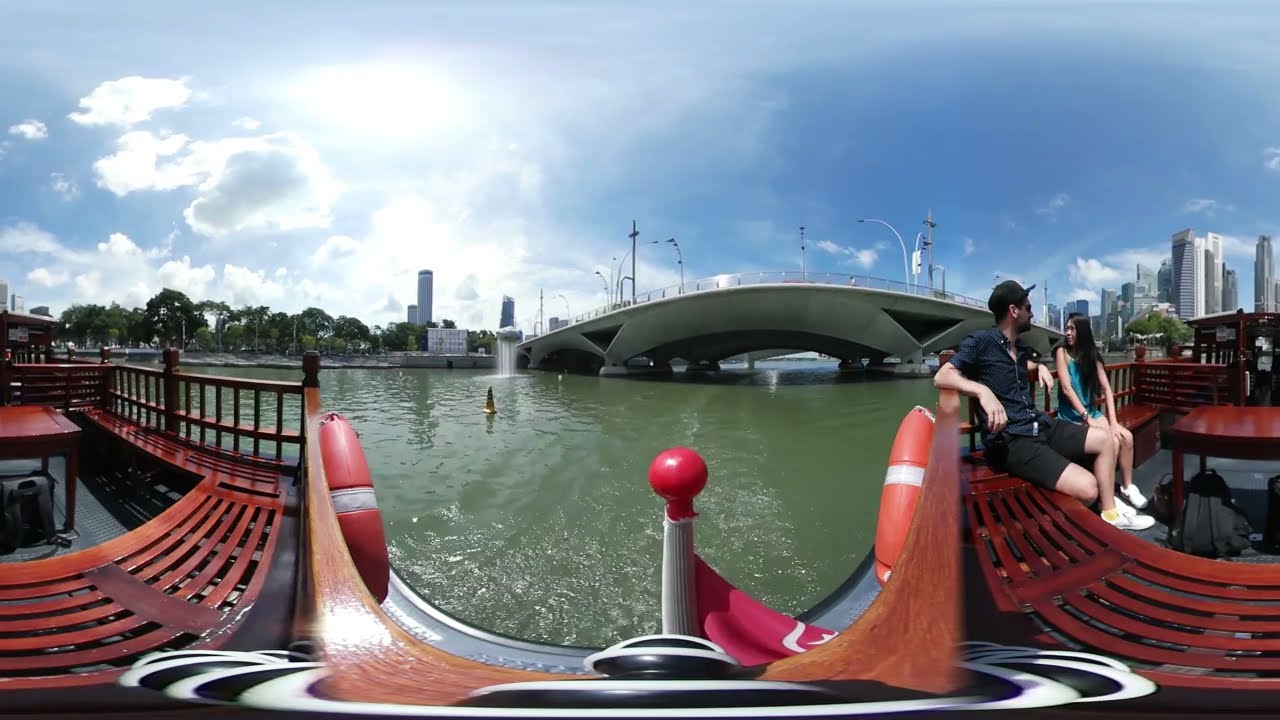This panoramic image, taken from a passenger ferry, showcases a scenic river tour through a major city. The ferry features charming cherry-red wooden benches and railings, enhancing its touristy, almost restaurant-like ambience. At the stern of the boat, a little red flag waves alongside a couple of lifesaver rings positioned at the railing. A young man and woman, possibly a couple or relatives, sit on the right-hand side bench. The man is dressed in a button-up short sleeve gray shirt and black pants, while the woman wears a blue tank top and has long black hair. The river, appearing slightly muddy and gray, winds through the city, bordered by lush trees and tall buildings. The boat is either about to pass under or has just emerged from a modern, curved bridge adorned with lights. Skyscrapers dominate the skyline in the background, with additional high-rises standing prominently on either side of the river. The scene is captured on a bright, partly cloudy day, adding depth and liveliness to the vibrant urban landscape.